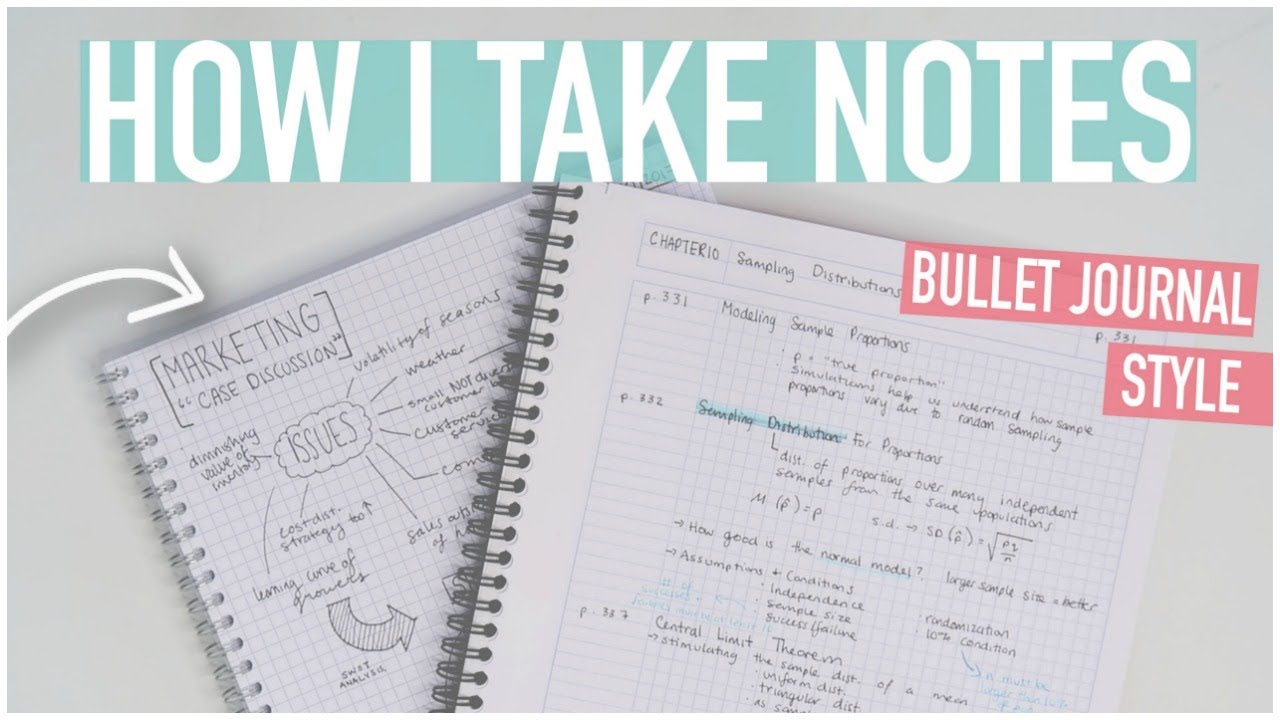The image depicts a photograph of a PowerPoint slide with a gray background, commonly seen as a blog header. At the top of the image, a bold heading in all-capital white letters set against a blue (possibly teal) background reads "HOW I TAKE NOTES." Below this heading and to the right, a subheading in white capital letters on a red (possibly pink) background states "BULLET JOURNAL STYLE."

Central to the image are two stacked notebooks, both featuring graph paper. The notebook on top is labeled "Chapter 10: Sampling Distributions," with page numbers for various sections highlighted in blue. This notebook includes more complicated math formulas and appears organized in a bullet journal style.

The notebook underneath is more prominently featured and illustrates a "Marketing Case Discussion." It contains the title "Marketing Case Discussion" and a diagram or flowchart outlining key issues such as the volatility of seasons, weather, and customer service. These issues branch out from a central idea labeled "Issues," depicted within a cloud-like shape with lines representing rays pointing to the respective text.

Additionally, a small white arrow with a drop shadow on the left side of the image directs attention towards the notebooks. This detailed representation serves to convey effective note-taking methods through organized and visually appealing styles.